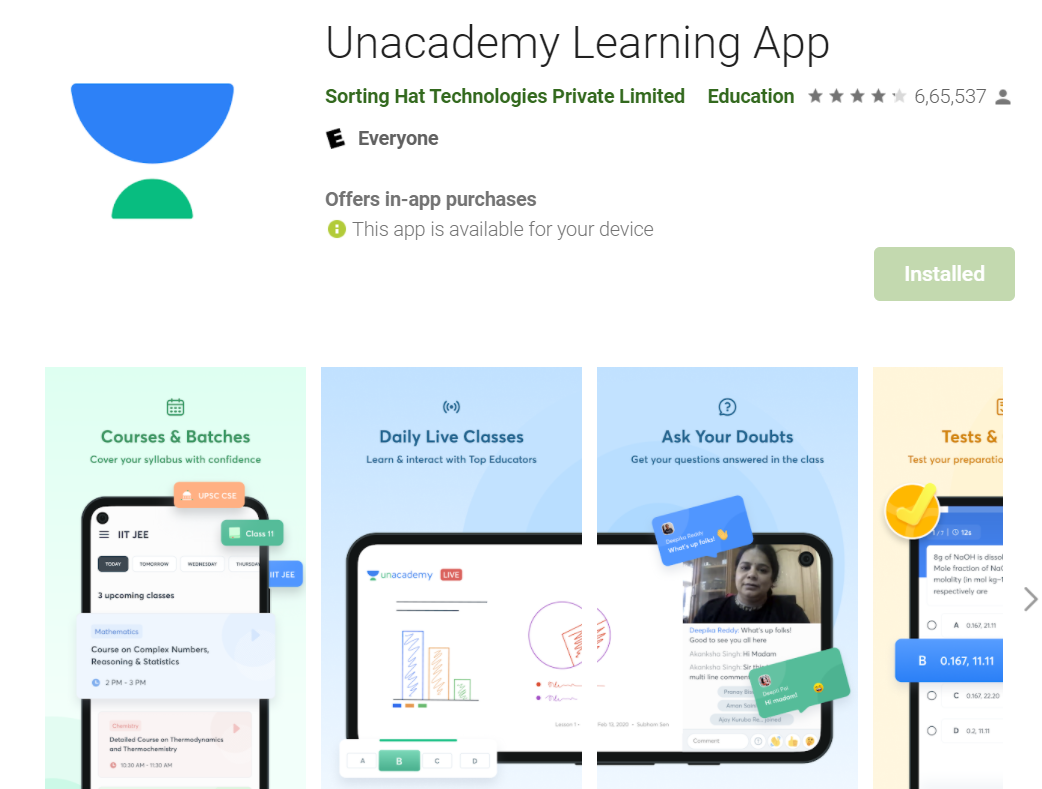This image is a detailed screenshot from an app store, though it is unclear whether it is from Google Play or the Apple App Store due to the absence of specific identifiers. The background of the screenshot is primarily white.

At the very top, the app name, "Unacademy Learning App," is displayed in a thin gray font. Below that, in a slightly darker gray font, the developer's information, "Sorting Hat Technologies Private Limited," is listed, followed by the category "Education."

The app boasts a commendable rating of 4 stars out of 5, supported by a substantial number of reviews totaling 665,537. To the left, the app is marked as suitable for "Everyone," and there's a note indicating that it offers in-app purchases. Additionally, it mentions that the app is available for the user's device.

The app icon is visually distinctive, featuring a blue half-circle resembling a bowl with a vertical line at the top. Beneath this blue bowl shape is an inverted green half-circle, about half the size of the blue one.

Below the icon, the screenshot provides a glimpse into the app's features, organized in rectangular sections with very light backgrounds. The first rectangle, with a light green hue, is titled "Courses and Batches," accompanied by an unreadable screenshot from the app. The next two rectangular sections are light blue, labeled "Daily Live Classes" and "Ask Your Doubts," respectively. Lastly, there is a landscape-mode screenshot showing a black and white photo of an Indian woman with dark hair in the upper right-hand corner. She is wearing a dark shirt, adding a personal touch to the app's promotional materials.